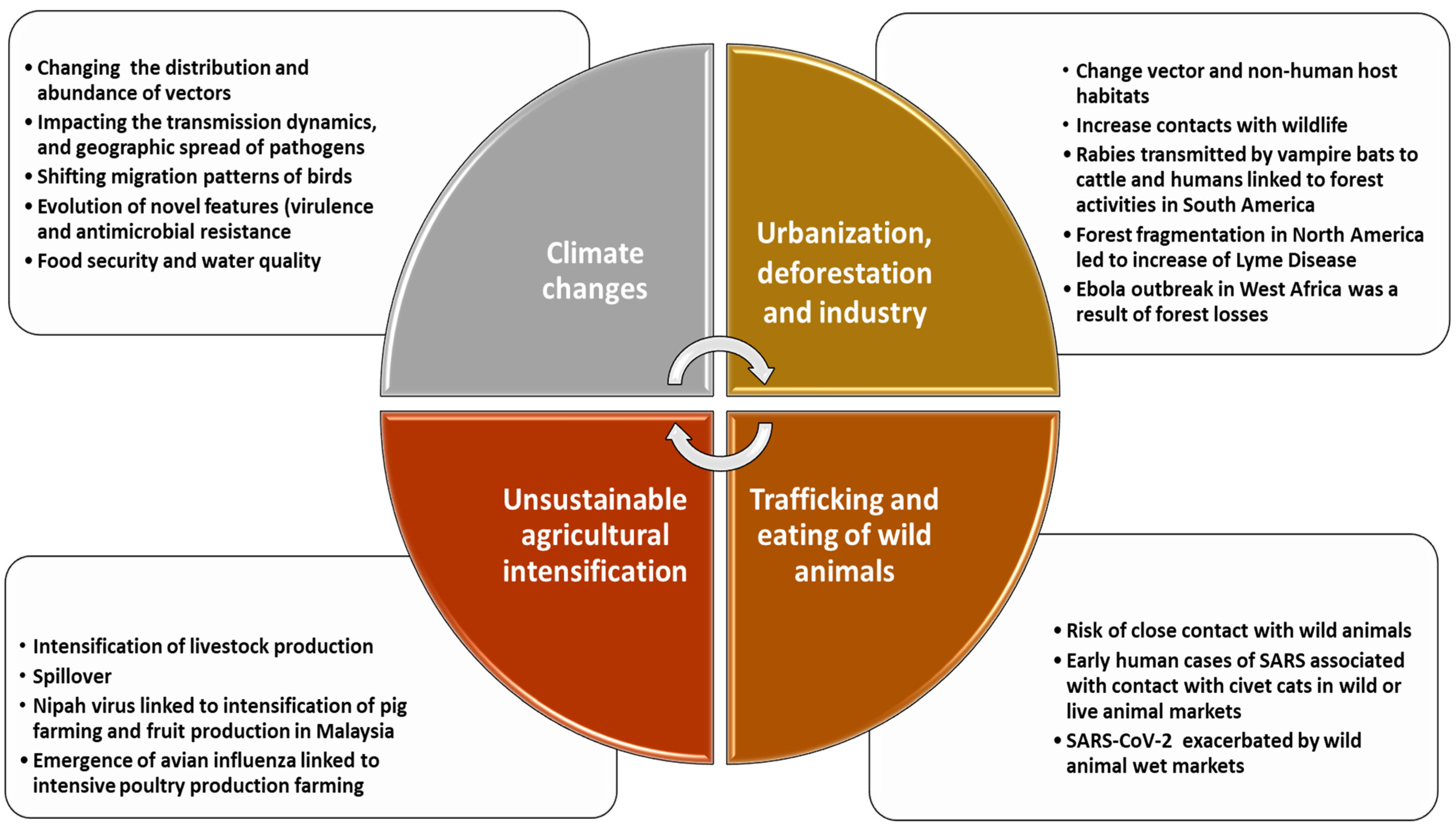This illustration presents a detailed breakdown of various environmental and societal factors impacting global health. At the center, a circle is divided into four equal quarters, each distinguished by color and topic. The upper left quarter, shaded in gray, is labeled "Climate Changes" and includes detailed bullet points on changing vector distributions, altered transmission dynamics of pathogens, shifts in bird migration patterns, evolution of novel features, virulence, antimicrobial resistance, and impacts on food security and water quality. Moving clockwise, the upper right quarter is brown and addresses "Urbanization, Deforestation, and Industry," indicating the impact of these human activities. The bottom right quarter, in a darker brown, is dedicated to "Trafficking and Eating of Wild Animals," highlighting issues related to wildlife trade and consumption. Finally, the bottom left quarter is reddish, and focuses on "Unsustainable Agricultural Intensification," underscoring the challenges of intensive farming practices. Surrounding each segment are rectangular boxes with a thin black outline, each containing bullet points that delve deeper into these topics. In the center of the circle, two arrows illustrate a clockwise cycle, showing the interconnectedness of these issues.